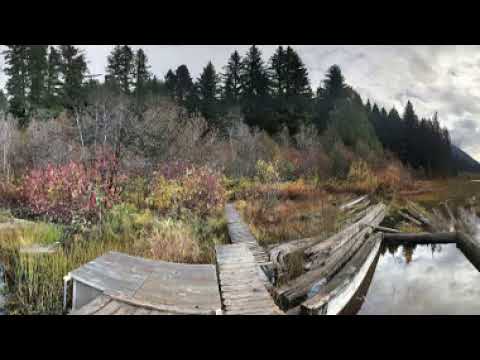The image presents a serene, nature-based scene featuring a lush, grassy foreground with scattered red leaves. Prominent in the foreground is a weathered, likely broken dock, its pieces strewn about amid the grass and plants near the small body of water, possibly a pond or lake. The water itself is barely visible, peeking out from behind the dock. The midground reveals a mixture of bushes and tall grass, appearing more colorful as they approach the viewer, with shades of green, tan, pink, orange, red, and gray. Large, dark green trees stretch across the background from left to right, while a range of mountains is visible on the image's right side. The top section of the image displays an overcast sky, heavily blanketed with clouds, suggesting a cloudy day in the middle of a tranquil, outdoor setting. The overall scene has a calm, untouched, and almost abandoned feel, accentuated by the absence of people and the natural dilapidation of the dock.